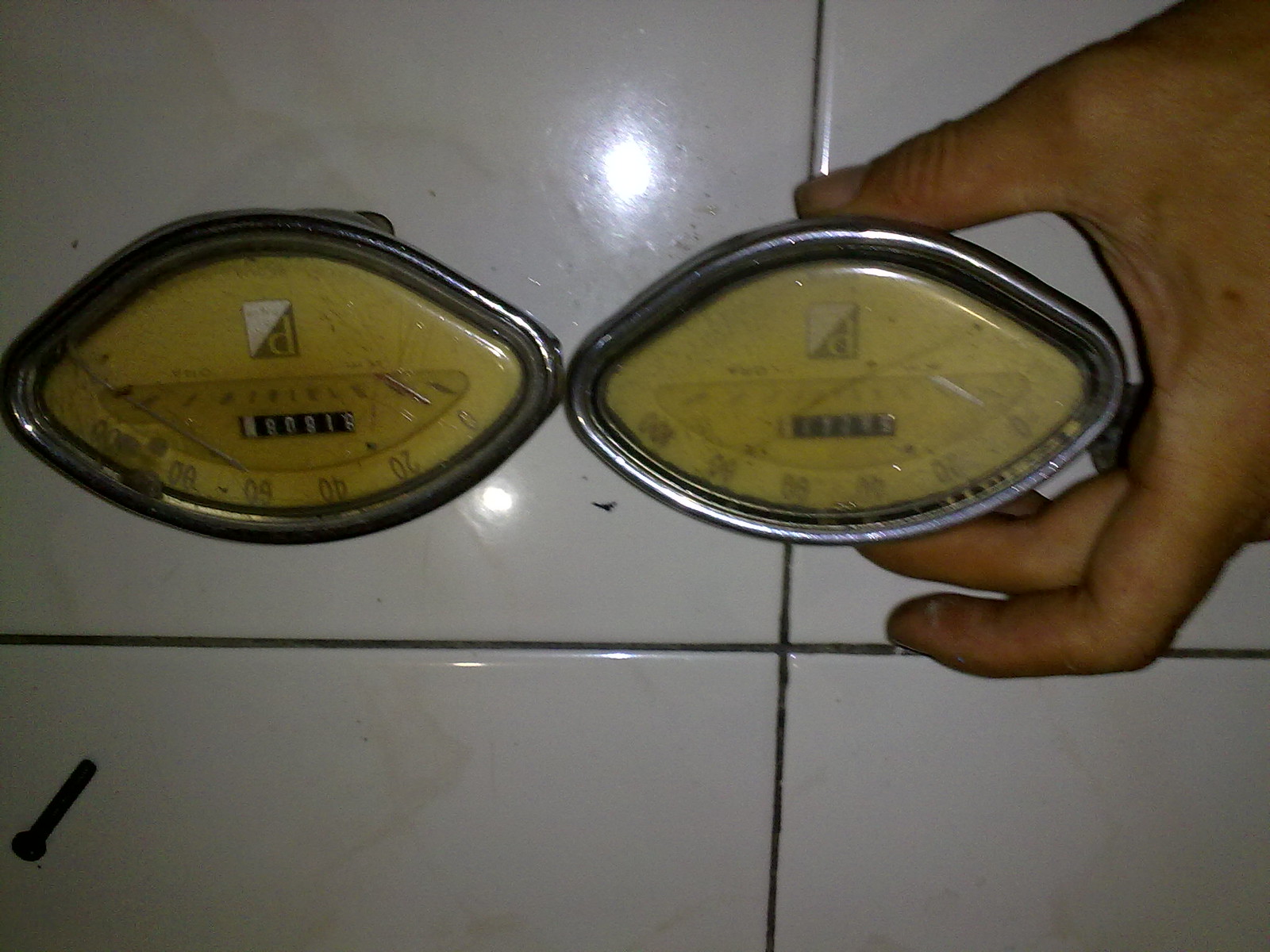This photograph showcases two antique, eye-shaped speedometers, positioned upside down on a glossy white tile floor with dark grout. The left speedometer is sharper in focus compared to the slightly blurred right one, potentially due to the camera's focus or the fogged glass on the latter. A rusty, approximately two-inch long bolt lies in the lower left corner of the frame. A hand, partially visible, reaches in from the right, holding the less focused speedometer. Behind the glass face of each speedometer is a yellowed background displaying the usual readings, ranging from 0 to 100. At the bottom of each device, an upside down, split rectangle logo in black and white features a prominent "P" in the black section, hinting at the maker’s brand. The intriguing composition offers a glimpse into vintage automotive instrumentation against a modern tiled backdrop.